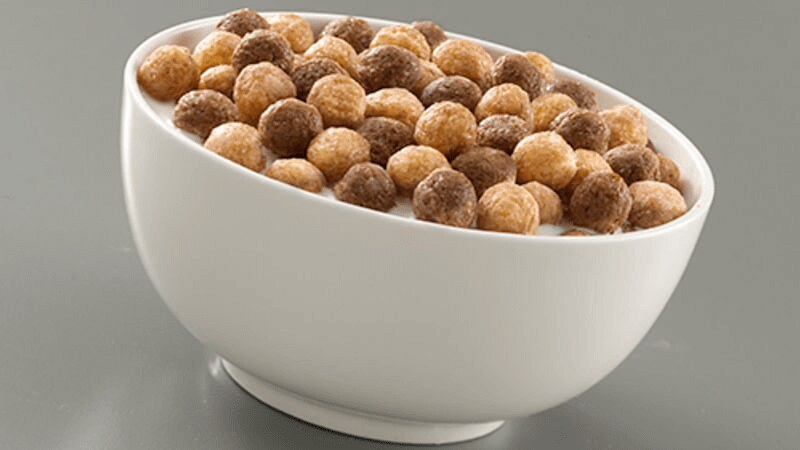In this image, a white deep dish bowl filled to the brim with Reese's Puffs cereal sits on a shiny silver or stainless steel surface. The cereal, consisting of round puffy balls in chocolate brown and peanut butter brown hues, is floating in milk, which can be seen on both the left and right sides of the bowl. The entire setup is slightly tilted to the right, giving the impression that the bowl is at an angle. The background’s reflective quality highlights the bowl's contents and adds a modern, sleek touch to the overall scene.